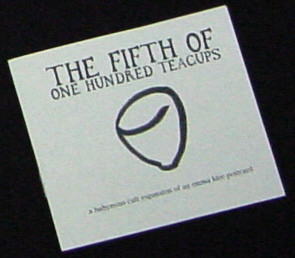The photo features a square white book placed diagonally at about a 30-degree angle against a stark black background. The cover of the book prominently displays the title "THE FIFTH OF 100 TEACUPS" in all capital letters, with "THE FIFTH OF" written in a larger old-fashioned serif font than "100 TEACUPS." Just below the title, there's a hand-drawn image of an upside-down triangle, resembling a crude teacup without a handle, outlined in dark black. At the bottom of the cover, there's a small, nearly illegible subheading that adds an element of mystery. The overall minimalist design focuses attention on the book's cover and the intriguing snippets of text it bears.